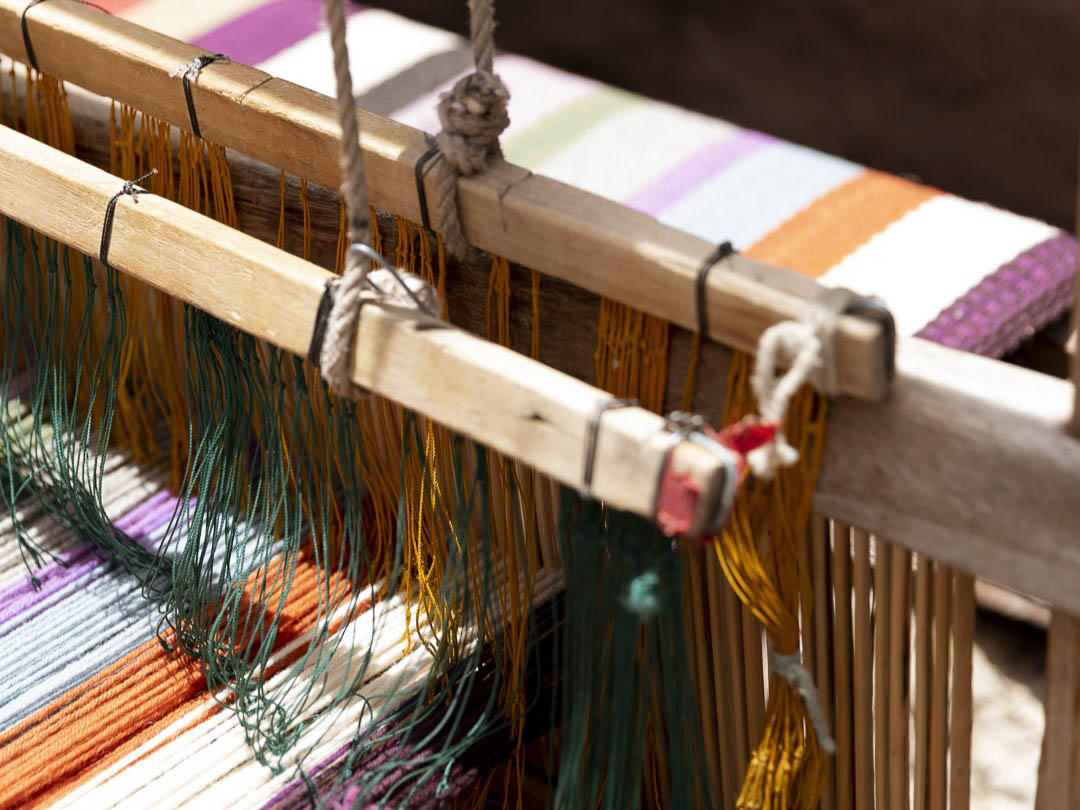This detailed close-up color photograph captures a loom in the process of weaving a vividly striped fabric. The background is black, providing a stark contrast to the vibrant colors in the frame. The loom features a wooden bar running from the upper left to the middle right, with multicolored threads suspended below it. The woven fabric showcases a sequence of stripes in royal purple, white, orange, baby blue, lilac, light green, and black, with the pattern repeating. Several smaller wooden dowels hang from the loom, with strings in various colors tied with a white piece of rope above. This loom is meticulously set up for creating what could become a beautiful and colorful blanket or scarf.